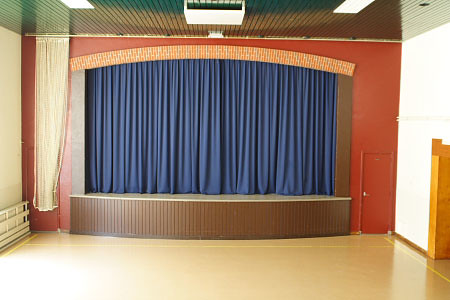The image captures an empty indoor theater stage, photographed head-on from a standing, eye-level position. The stage floor is made of light-colored, shiny wood, enhancing the room's spacious feel. The lower front of the stage features a brown wooden frame, while the stage’s upper section and sides are painted in a rust color. The central stage is flanked on both sides by doors, with the walls painted in a cream and white pattern. A dark blue curtain lines the back of the stage, with an additional ivory-colored curtain pulled to the side. Overhead, wooden paneling adorns the ceiling, interspersed with visible lighting fixtures. The space suggests a multifunctional room, likely a small theater or school playroom, bathed in natural light filtering through unseen windows.